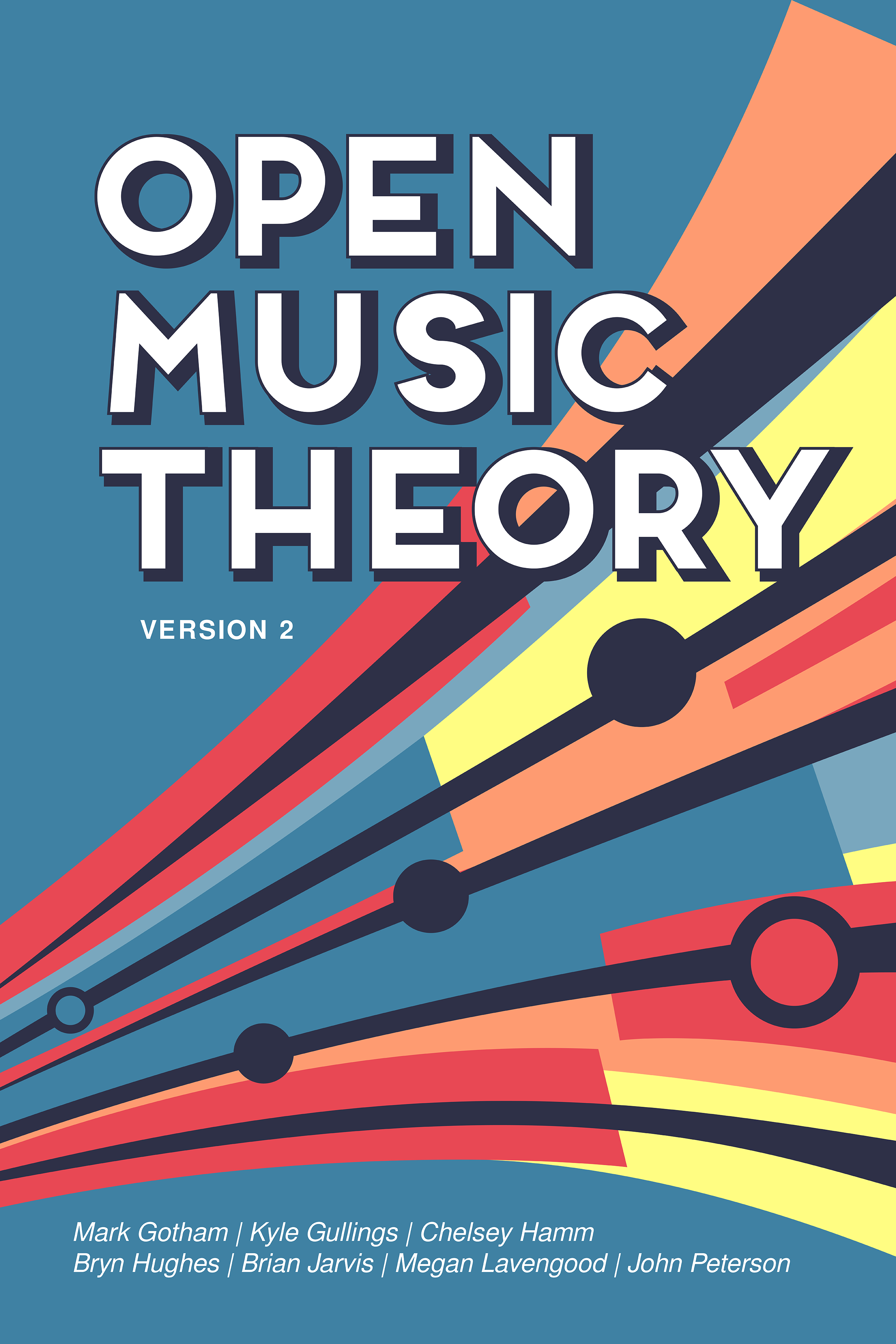The cover of the book, titled "Open Music Theory: Version 2," features a vibrant and abstract design sweeping from left to right. Set against a blue background, the cover is adorned with five colorful curves resembling sheet music, incorporating red, orange, yellow, blue, and black hues. Among the curves, there are circles symbolizing whole notes and open circles representing half notes. The title is prominently displayed at the top in big, bold white letters outlined in black. The authors, listed in white lettering at the very bottom, include Mark Gotham, Kyle Gullings, Chelsea Hamm, Brian Hughes, Brian Jarvis, Megan Lavengood, and John Peterson. This dynamic cover suggests a lively exploration and celebration of music theory.